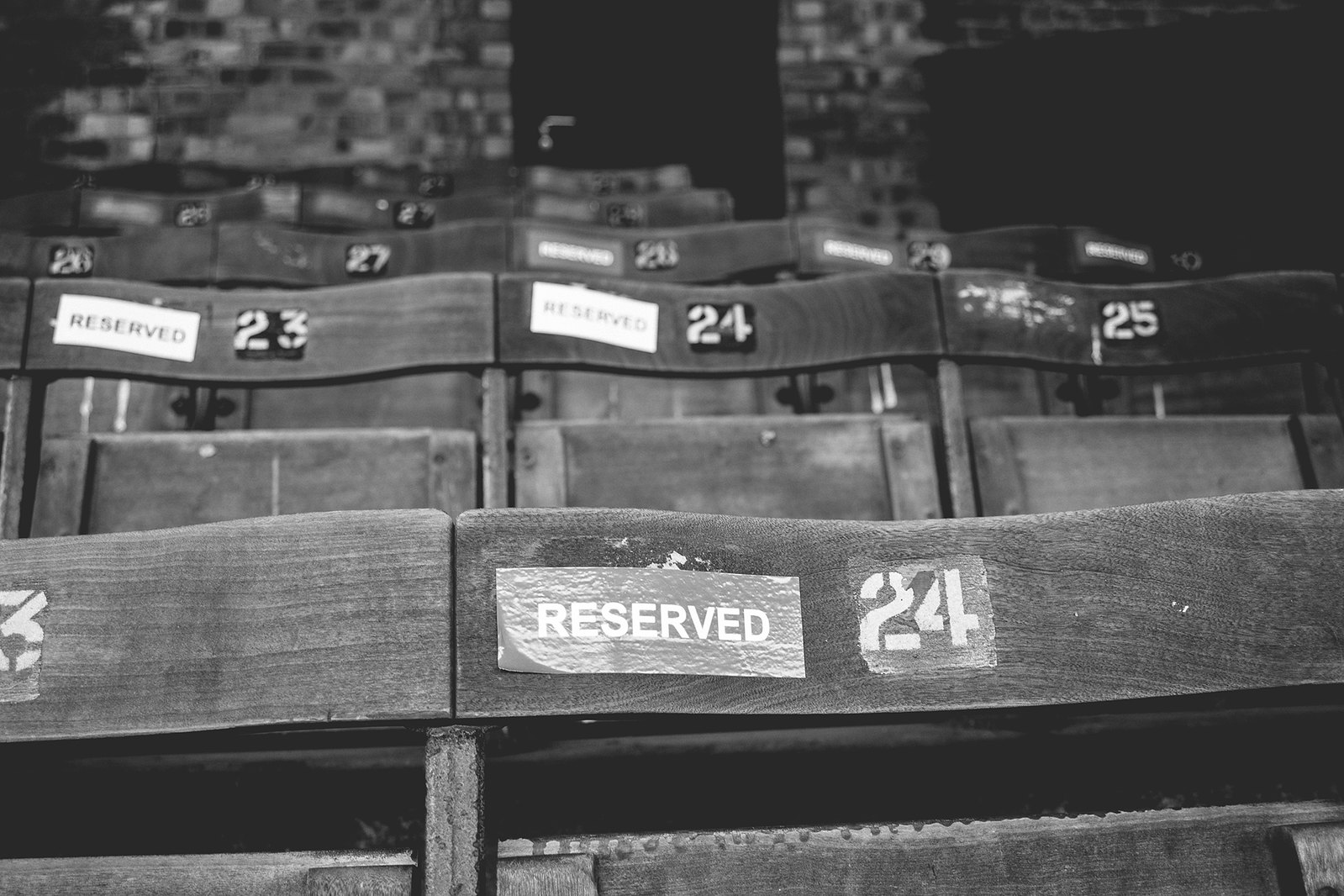The black and white photo captures an older auditorium or stadium with multiple rows of wooden folding chairs. In the foreground, a sign reading "Reserved" and marked with the number 24 is prominently displayed. The row behind it features chairs numbered 23, 24, and 25; both 23 and 24 have white "Reserved" signs, while chair 25 appears to have its sign missing or torn off. Further back, another numbered row includes chairs labeled 26 through 30, with "Reserved" signs on 28, 29, and 30, while chairs 26 and 27 do not have any designation. The photo's depth fades into blurred rows of additional chairs that can't be distinctly seen. The setting is partially illuminated, giving the room a dim, vintage atmosphere. The chairs, with their curved wooden backs, appear worn and aged, possibly from the 1950s, not shiny or lacquered but well-used. In the background, a brick wall with a central black doorway can be seen, with parts of the wall flat and devoid of bricks, suggesting a combination of brickwork and drywall.